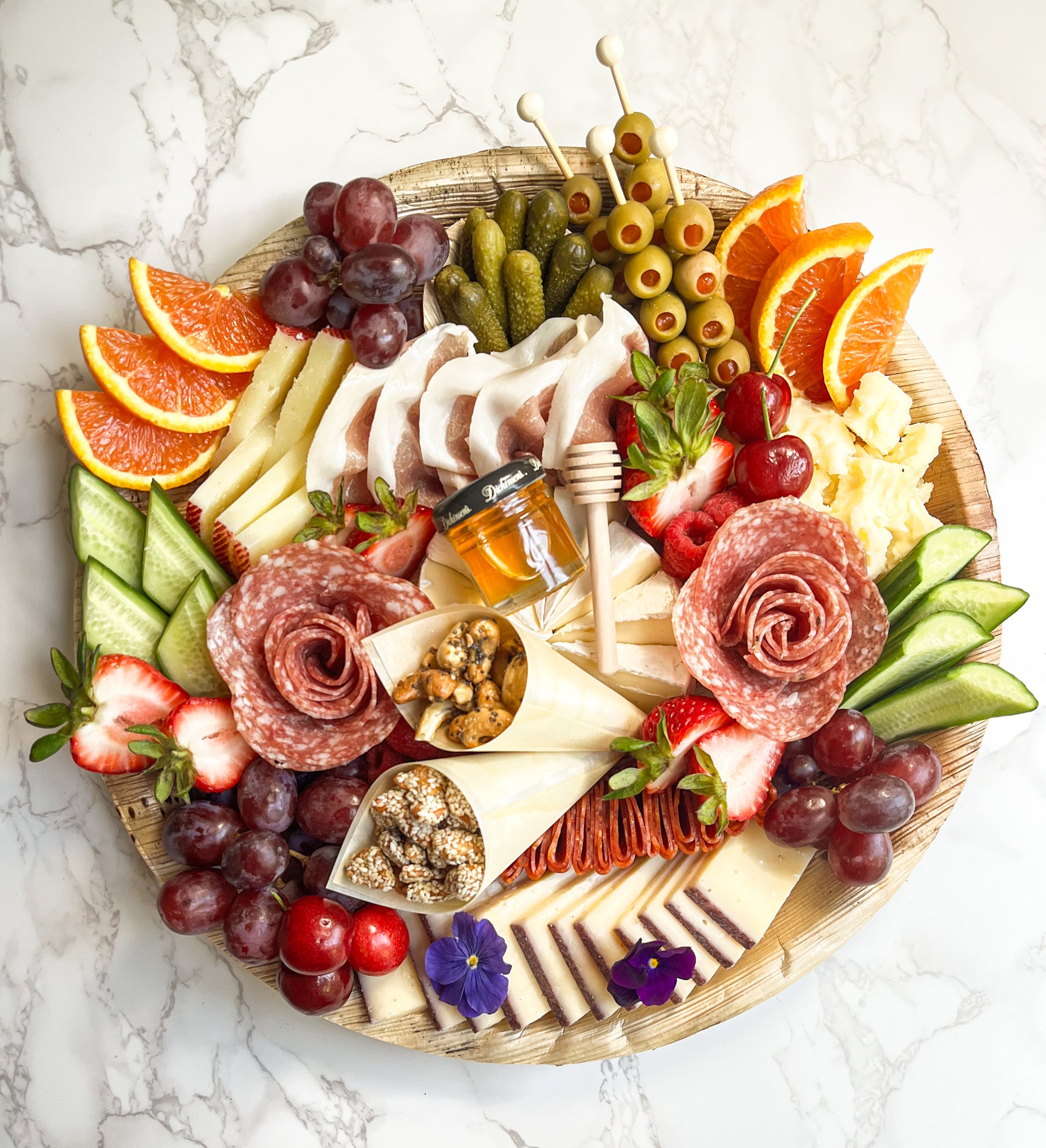In this top-down photograph of a charcuterie board, we see a beautifully arranged wooden platter resting on a white granite countertop streaked with gray. The board features a delightful variety of foods. At the center, there's a wedge of brie cheese topped with a honeycomb dipper and a jar of honey. Surrounding this are green olives with pimentos on skewers, small pickles, red grapes at the bottom, and neatly sliced cucumber sticks. There are two elegant salami rosettes and some prosciutto, along with two types of cheese, one adorned with purple flowers. Brightly colored fruits add to the visual appeal, including sliced strawberries on the left, orange slices, a few cherries, and scattered raspberries. Nuts covered in toffee can be found near the center, and dark blue flowers provide decorative touches around the platter, making it as visually appealing as it is appetizing.